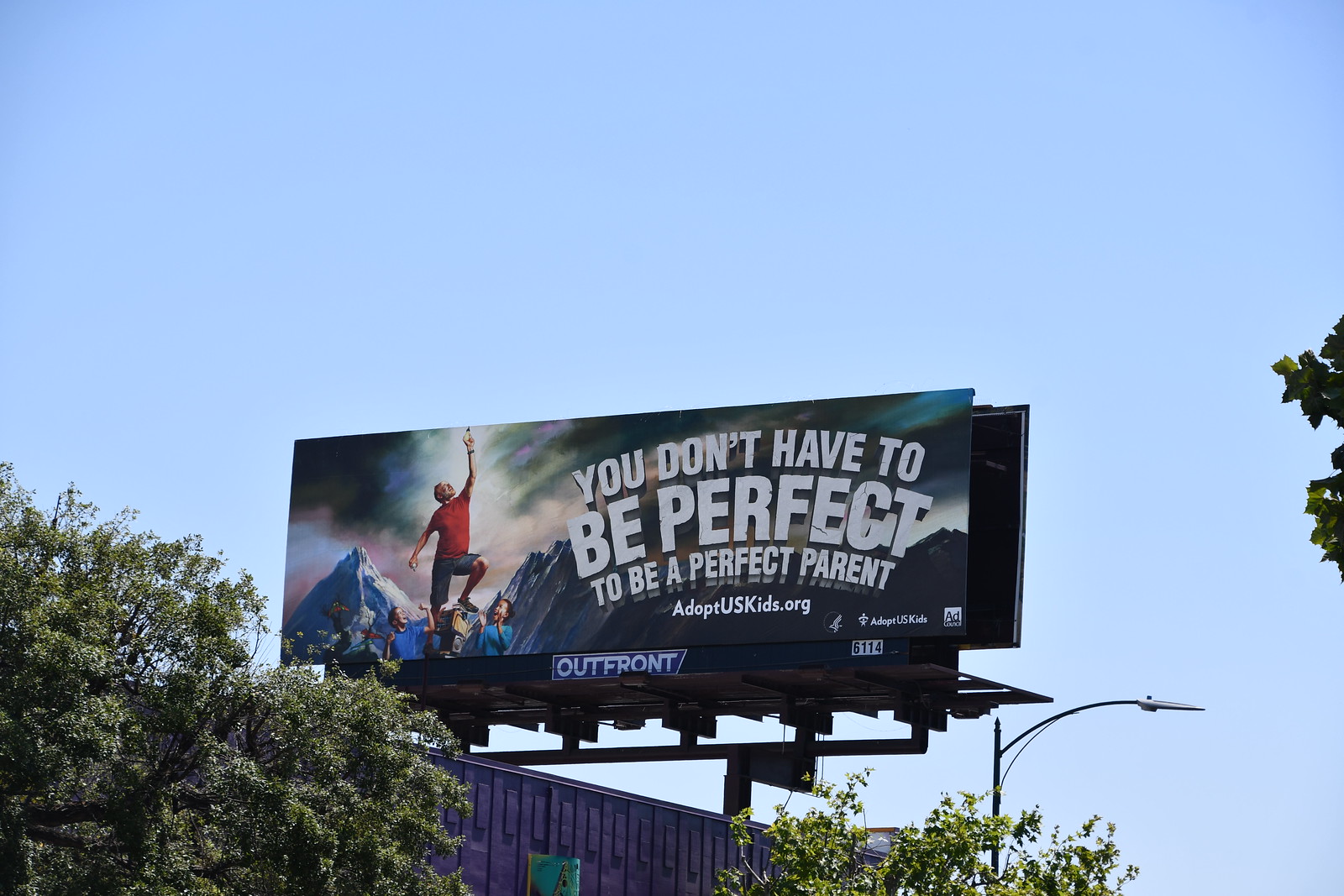This photograph features a detailed view of a billboard prominently mounted on top of a purple building, with sections resembling a gray bridge supported by two tall legs and adorned with a green traffic sign. The scene is framed by several deciduous trees, situated on the left, beneath, and to the right of the billboard, with their crowns visible against a clear, blue sky. The billboard itself depicts a man in a red t-shirt and possibly cut-off jeans, standing triumphantly, supported by three others—two in blue shirts—against a backdrop of jagged mountains. The man, wearing a wristwatch, raises a hand to touch the top of the sign. The upper part of the billboard is dominated by dynamic, curving white text that reads: "You don't have to be perfect to be a perfect parent," followed by the URL, "AdoptUSKids.org." The billboard is operated by Outfront, indicated by their logo and the number 6114 at the bottom. This powerful advertisement underscores the message of the triumph and joy found in adopting children.